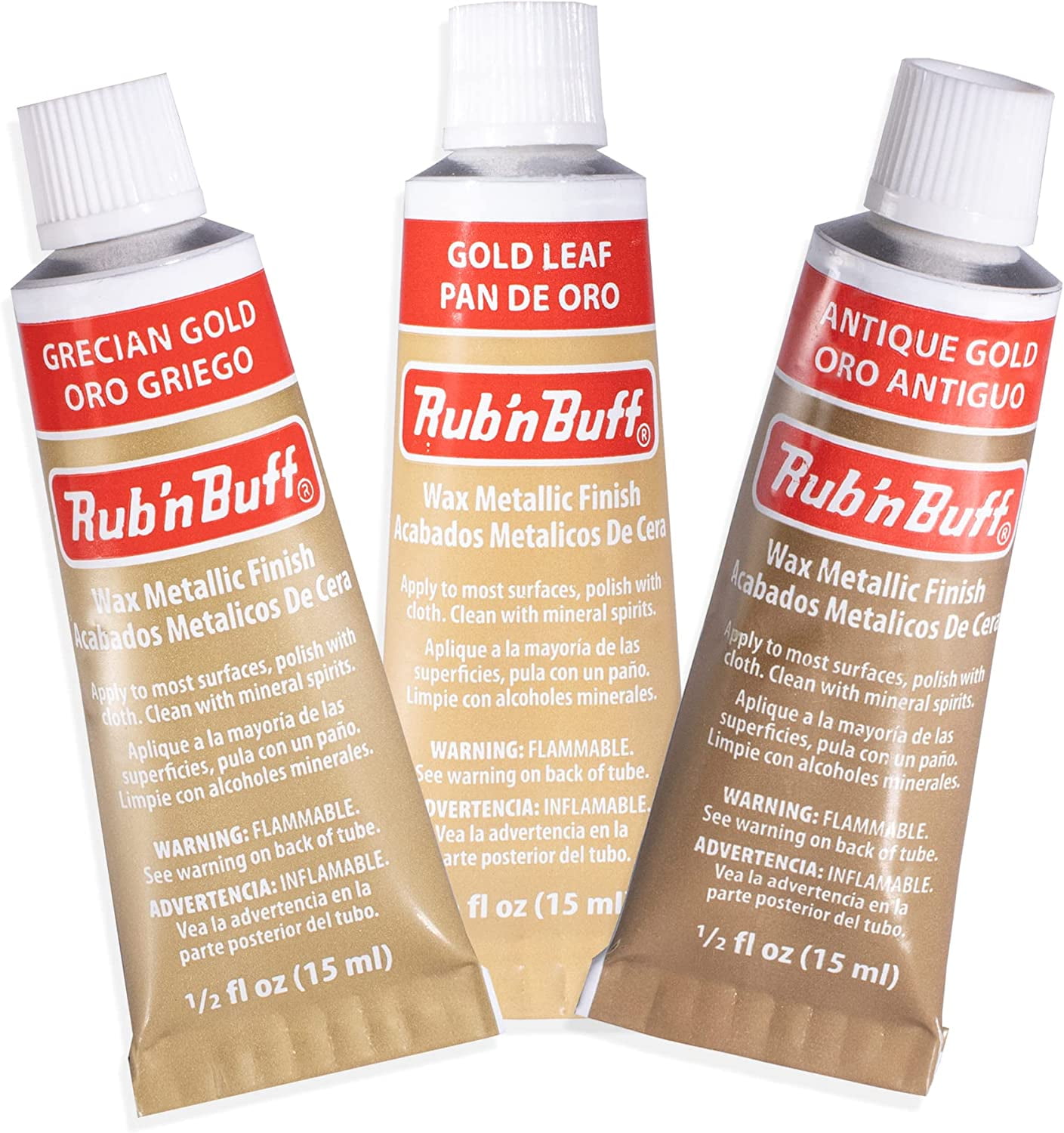The product image showcases three tubes of Rub and Buff wax metallic finish, arranged on a white background. The central tube stands upright with its white cap facing the camera, labeled "Gold Leaf" with the Spanish translation "pan de oro." Flanking it, two tubes are tilted at approximately 20-degree angles: the one on the left, angled to the left, is labeled "Grecian Gold" with "oro griego" underneath; the right-leaning tube is labeled "Antique Gold" with "oro antiguo." All tubes feature an orange strip indicating their color, metallic bronze bodies, and the Rub and Buff red rectangular logo. Additional text on each tube includes usage instructions in English and Spanish, a warning about flammability, and their volume of 0.5 fluid ounces (15 milliliters).